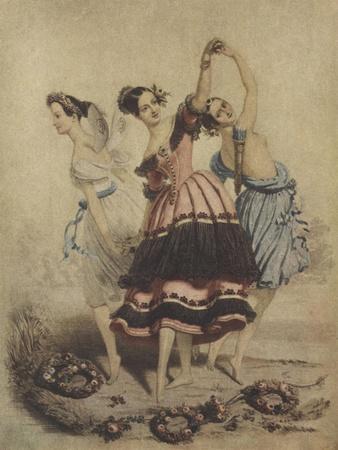This image depicts an old painting, possibly from the late 1800s to early 1900s, featuring three women who appear to be dancing gracefully, reminiscent of ballerinas. Their delicate hairdos suggest significant care, indicating an era where personal appearance was highly valued despite the challenges of the time. The women are barefoot and poised on their tippy toes, adding to the impression of a ballet scene. 

They are adorned in flowing, flower-like dresses: one in a light blue dress, another in a purple and pink dress, and the third in a white dress with a blue accent around her waist. The woman in the pink dress holds the hand of the woman in the blue dress, while the third woman stands apart. At the bottom of the image, there are three laurel-like shapes in shades of brown and light pink. The background features an off-white, almost yellowish hue with subtle hints of gray, adding to the antiquated charm of the piece. The dominant colors in the painting are pink, purple, blue, white, and gray, and there is no accompanying text.